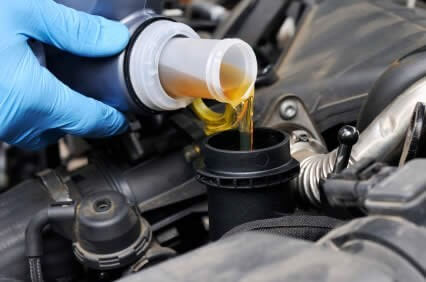The image depicts someone, partially visible with a gloved hand clad in blue latex, pouring a gold-brown liquid, presumably oil, into a component of a car engine. The oil flows from a blue bottle with a long rim into a black tubular opening. The engine area is marked by various mechanical parts predominantly in black with steel or silver detailing. The scene is a meticulous mix of gray metal car parts and visible gears, with additional black and silver components, creating a highly mechanical atmosphere. The liquid appears thick, pouring slowly, suggesting it is indeed oil. The setup indicates a routine maintenance task, likely prepping the car for use.